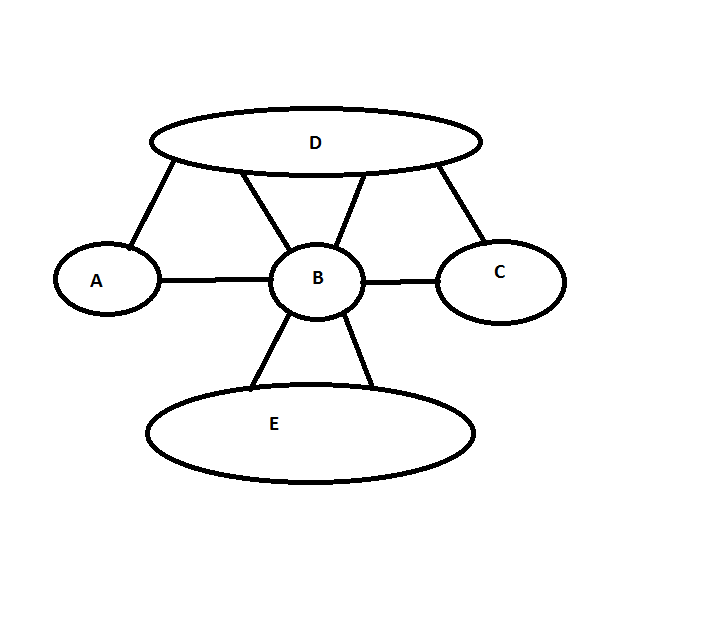This diagram illustrates the step-by-step assembly instructions for a piece of furniture, likely a coffee or cocktail table. The diagram contains five labeled sections (A, B, C, D, and E), each designated with distinct shapes and positions to clarify the construction process. 

- "A" is highlighted within an oval and connected to "D" through arrows, suggesting a pivotal attachment or alignment for these components. 
- "B" is centered and marked within a circular shape.
- "C" is denoted within a larger oval.
- "E" is positioned at the bottom in a wider, circular form.
- "D" is similarly represented within a wide circle.

The overall arrangement of these labeled parts forms makeshift triangles, aiding in visualizing the correct assembly sequence. This structured layout, combined with directional arrows, seems to guide the assembler in fitting the pieces together accurately, contributing to the table's unique features.